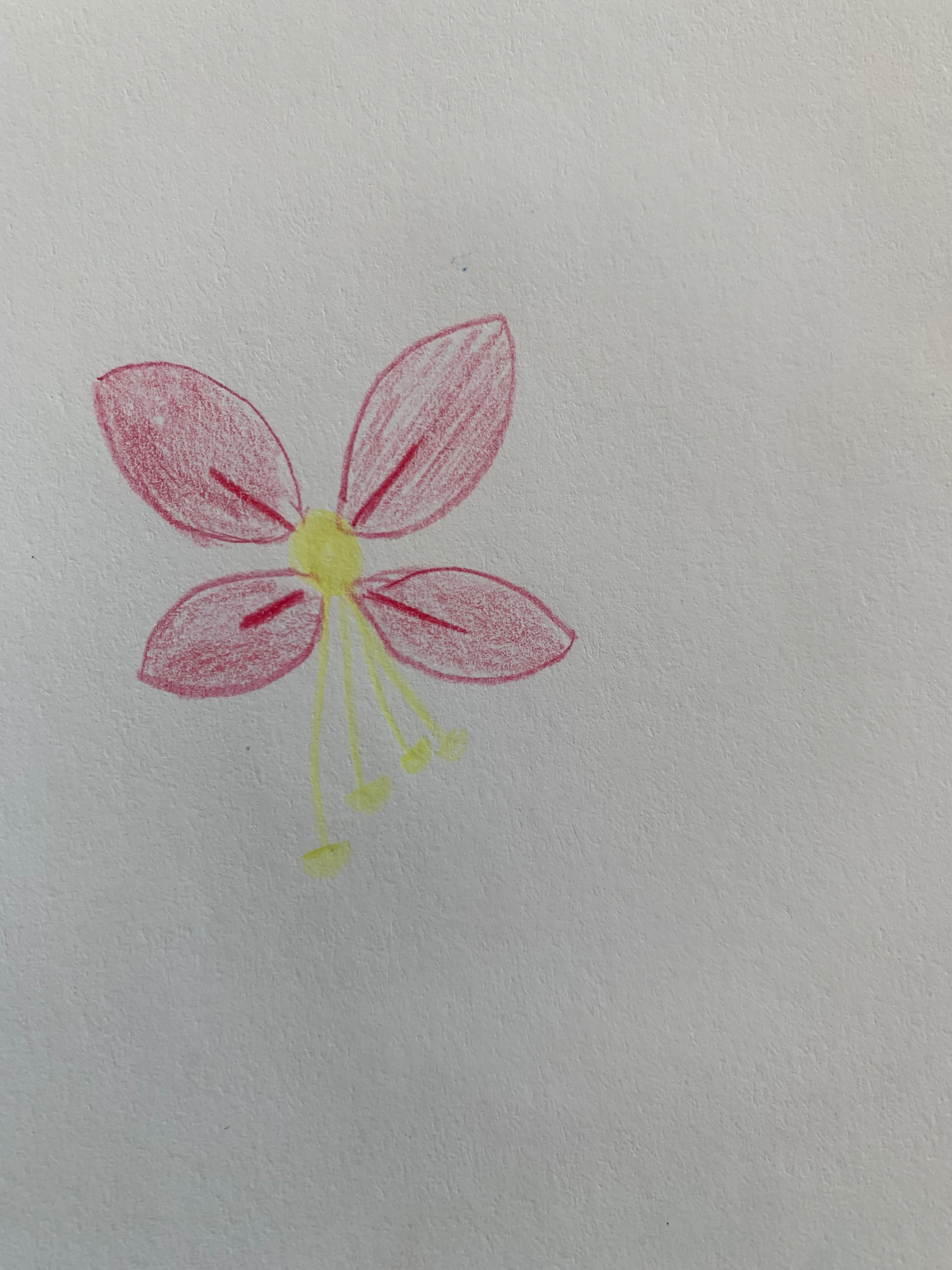This indoor color photograph showcases a textured piece of sketch paper that fills the entire frame. In the upper-left quadrant, slightly above the center, lies a simple yet charming crayon drawing of a flower. The flower features four large, oval petals, each outlined and shaded in shades of purple and red, with a darker line running halfway through the center of each petal, resembling veins. At the heart of the flower is a bright yellow circle, from which four yellow stamens extend downward, slightly veering to the right, each capped with small yellow dots of pollen. The overall composition is reminiscent of a child's drawing, characterized by its simplicity and lack of detailed intricacy, lending a charming, innocent quality to the artwork. There are no words, text, or print visible in the photograph.